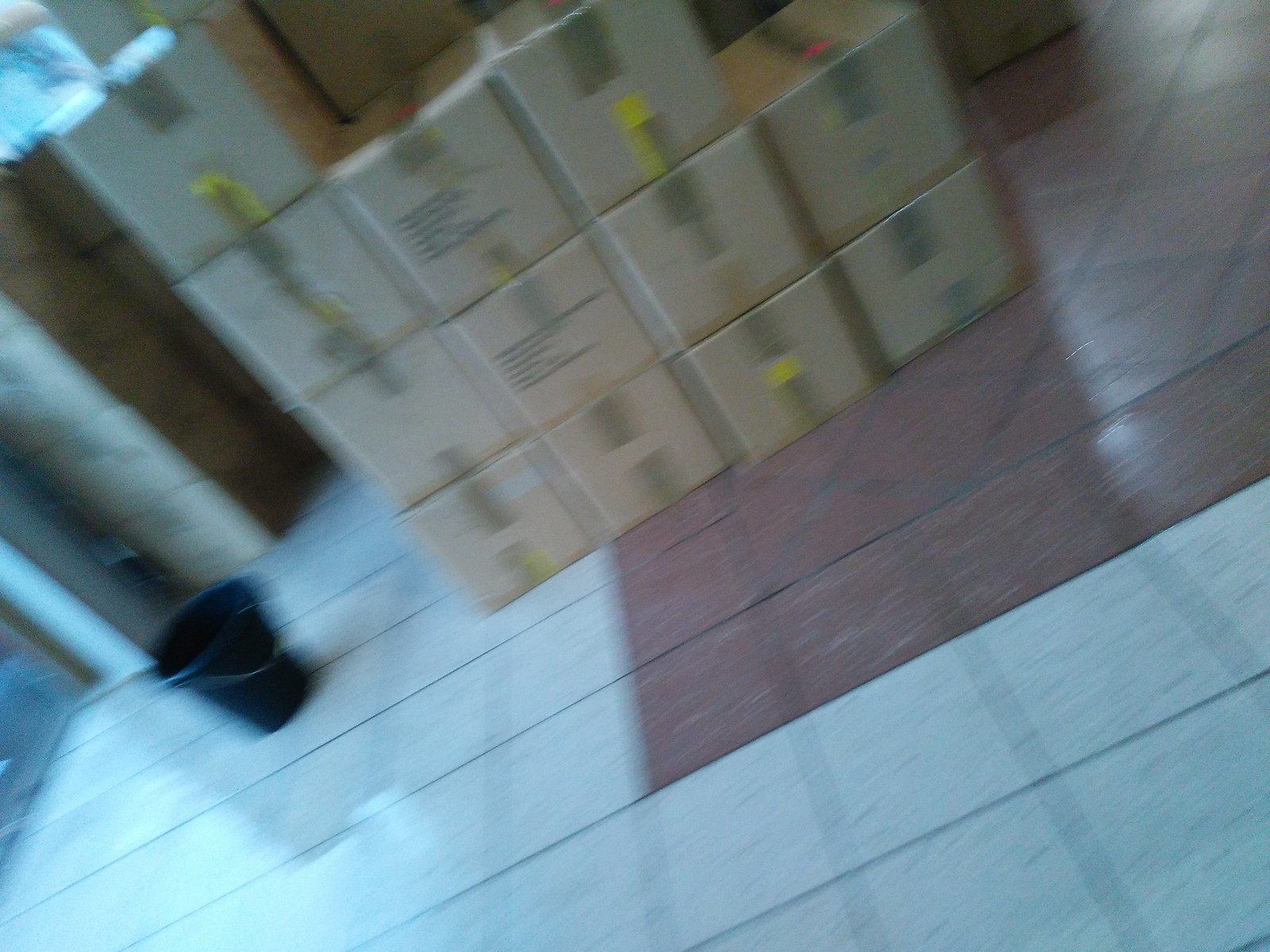This photograph, though quite blurry and grainy, depicts a collection of cardboard boxes stacked on top of each other on a tiled floor. The boxes are secured with yellow tape and feature black lettering. The floor is a mix of burgundy and off-white tiles with noticeable black grout lines. To the left of the stack of boxes, there is a black bucket with a silver handle positioned near a door. The light reflects off the tiled floor, adding a slight glisten to the scene. Portions of the door jamb are also visible, adding context to the setting.